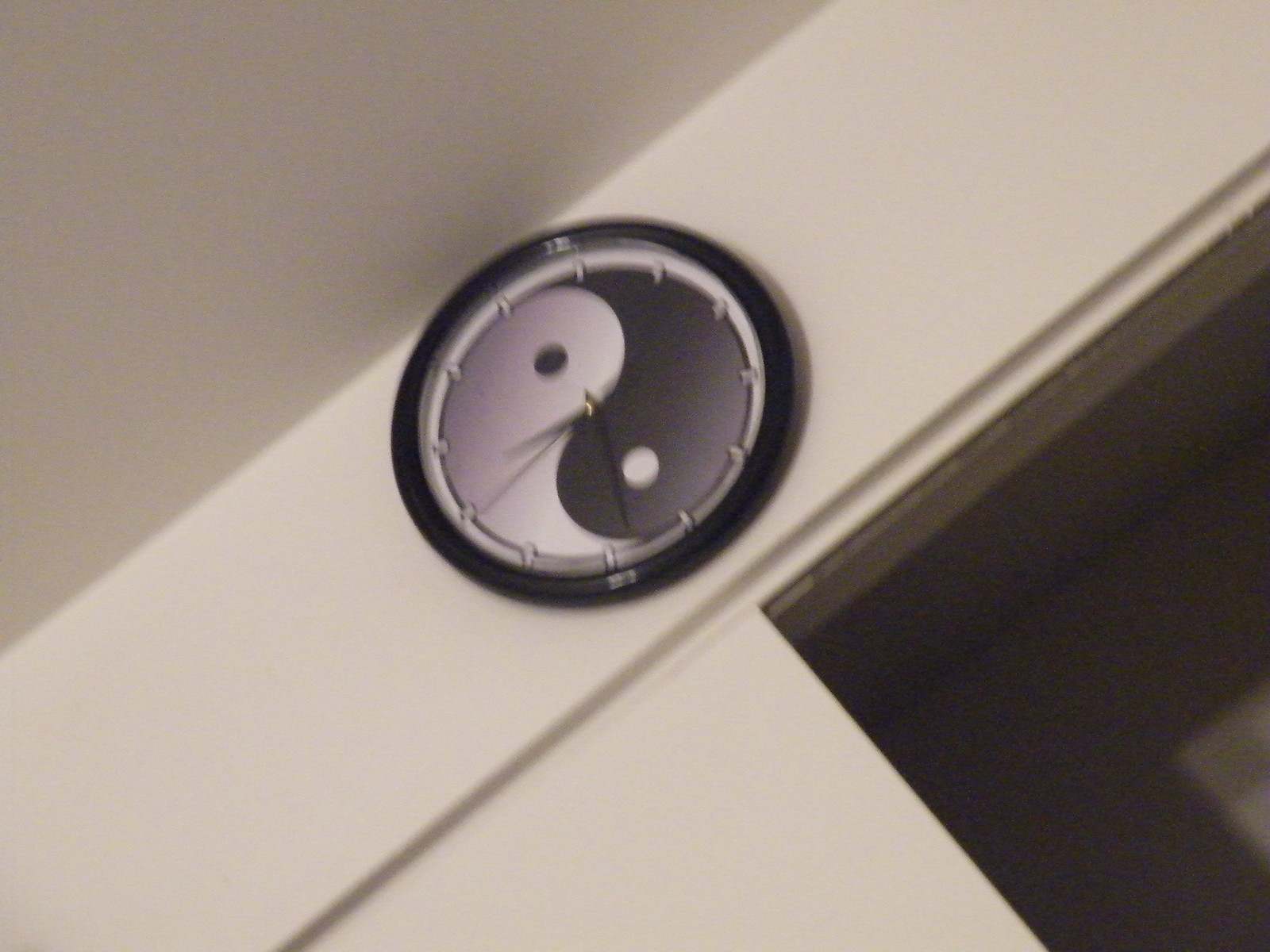This photograph showcases a large analog clock mounted high on an off-white wall, nearly touching the ceiling, above a dark doorway. The clock’s face features a distinctive yin-yang design, with the black housing framing a predominantly white interior interspersed with light gray accents. The yin-yang symbol extends diagonally across the clock, with the gray segment spanning from the bottom center to the top right and the black segment from the top center to the bottom left, forming a swirling circle. Each segment tapers off into a curved triangular shape, fitting together seamlessly like puzzle pieces. The white portion contains a black dot, while the black portion contains a white dot, representing the 'eyes' of the yin-yang. The clock hands—hour, minute, and second—are black, and the time displayed is approximately 9:34. Surrounding the clock face are small white hash marks indicating the hours, as there are no numerical digits present.